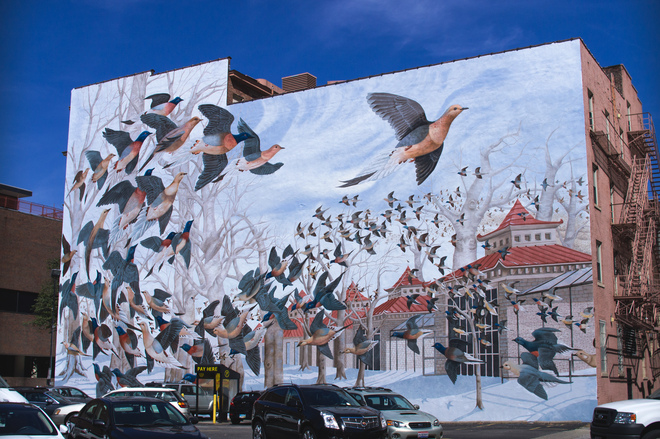This image captures the side of a four-story building adorned with a striking and detailed mural. The mural, set against the building’s light gray and cream-colored walls, vividly portrays a winter scene. Birds with white and blue feathers are depicted mid-flight across a sky dotted with clouds. Below the airborne birds, leafless trees stand against a backdrop of red-roofed houses that exhibit an Asian architectural style. The painted ground appears snow-covered, enhancing the winter atmosphere. Adjacent to this artwork is the right side of the building, featuring narrow windows and external stairs, painted in a pinkish-brown hue. In the foreground, several cars—white, black, and silver—are parked, suggesting a business area. The photograph, likely taken in the late afternoon or near sunset, captures a serene and artistic moment, with gentle lighting and a slightly blue sky overhead.